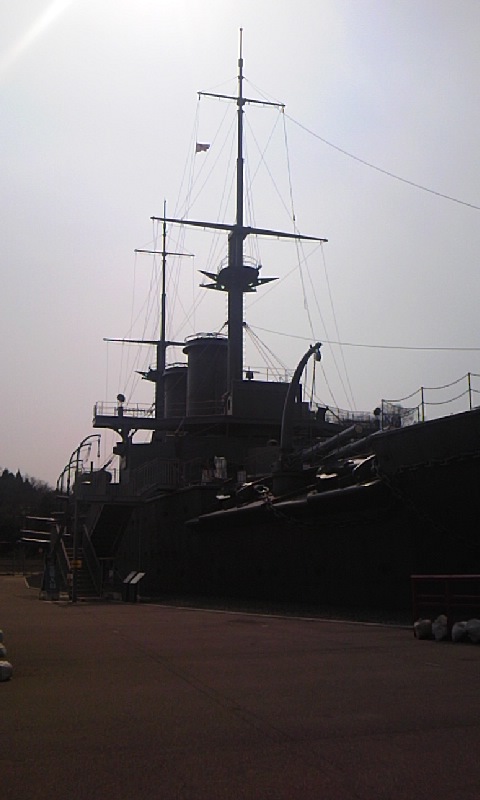The image captures a large, docked ship bathed in daylight, with the sun shining overhead, casting rays that illuminate the scene. The sky appears grayish-whitish, likely hazy. The ground below, paved with orange-ish, reddish, and dark brown hues, suggests an asphalt surface. The ship's imposing structure is fitted with multiple antennas, cables, and several tall masts with horizontal cross bars, giving an impression of a complex, well-equipped vessel. Prominent smokestacks rise from the deck, and various pillars and platforms, including a watchtower-like feature encircled by a railing, can be seen. The front of the ship showcases railings adorned possibly with chains, adding to its robust appearance. Steps are visible, leading up to the ship, indicating a point of access from the dock. In the distance, trees add a touch of natural scenery to the industrial backdrop, and a faint, white mark in the top left corner of the image, along with some blurred shapes, hint at further elements just out of clear view.